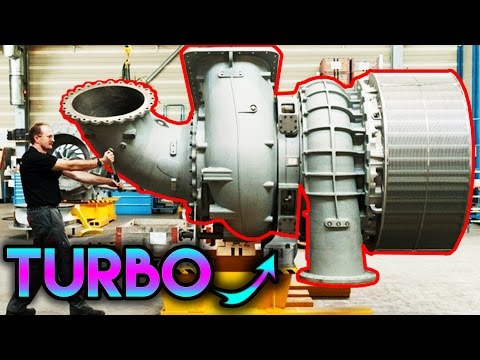The image showcases a massive turbocharger, taking up nearly the entire frame and outlined in a bold red border. The turbocharger, resembling the size of an airplane engine, dominates an industrial or warehouse-like setting with intricate silver piping and large cylindrical components. On the far left, a man wearing glasses, a black shirt, grayish pants, and black shoes, is seen holding onto a handle on the turbocharger, appearing tiny next to the colossal machine. In the bottom left corner, vibrant multicolored gradient text in blue, purple, pink, and teal boldly spells out "TURBO" with an arrow pointing towards the turbocharger. The image bears a black border on the top and bottom, giving it a designed, almost thumbnail-like appearance.